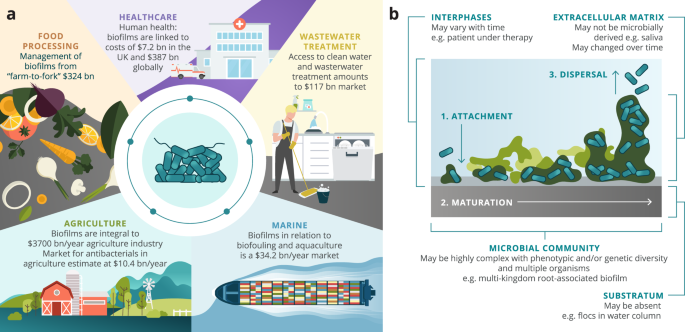This image features two detailed diagrams, labeled A and B, illustrating various aspects of biofilms and their impact on diverse sectors. 

Diagram A, positioned on the left, contains a central circle depicting bacteria cells that resemble blue capsules with black appendages. Surrounding this circle, in a counterclockwise pattern, are key areas affected by biofilms, including food processing, healthcare, wastewater treatment, marine biofouling, and agriculture. Accompanying this diagram are specific statistics such as the economic impact of biofilms: $7.2 billion in the UK and $387 billion globally, $117 billion for wastewater treatment, $34.2 billion in marine biofouling, and $3,700 billion in the agriculture industry. Also noted are terms like "interfaces," "extracellular matrix," "dispersal," and "attachment," highlighting various stages and components of biofilm development.

Diagram B, on the right, labeled with a lowercase "b," is described as science-related and includes a significant focus on the "microbial community." This section delves into more specifics about biofilm structures and their phases, such as the "extracellular matrix" and "maturation phase," illustrated in a colorful and animated style with bright hues of orange, green, and blue, indicating the scientific processes and stages of biofilm life cycles. 

This visual compilation seems to serve an educational purpose, possibly derived from a textbook or an informational booklet aimed at explaining the critical roles and impacts of biofilms across various industries.